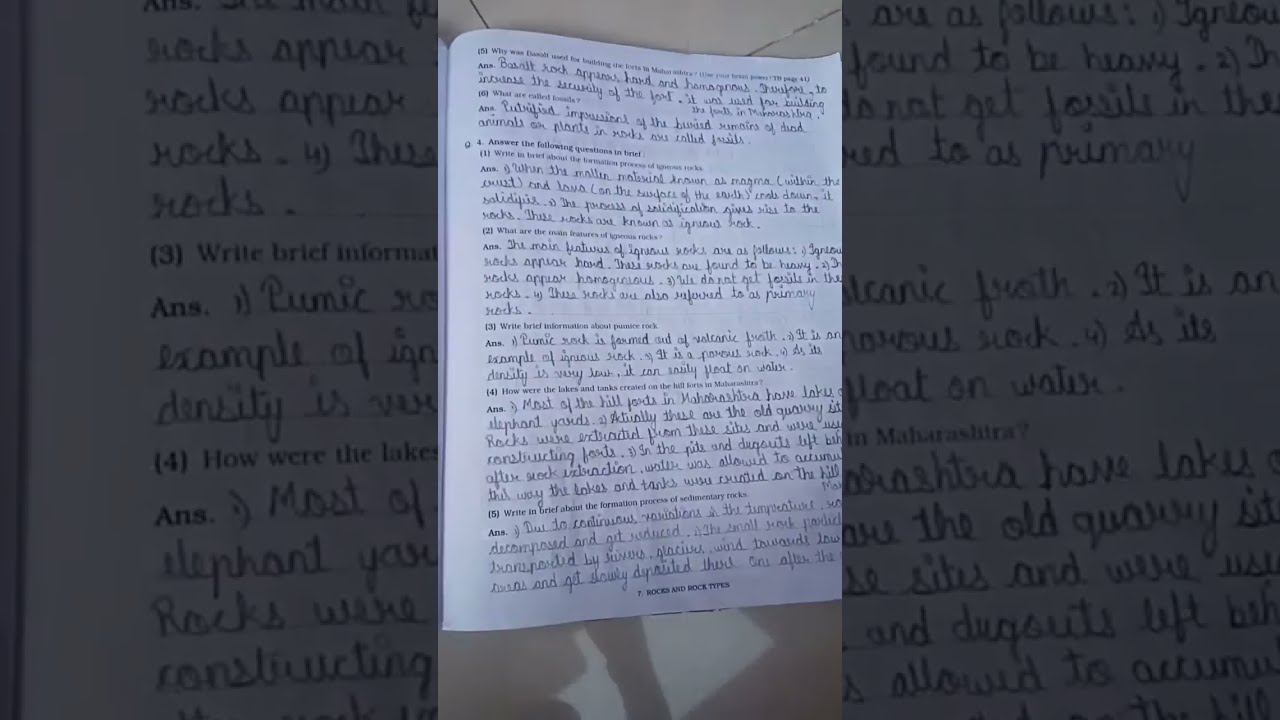The image is a photograph of an open booklet, likely a school test or textbook page, centered on a tiled floor. The page is densely populated with questions and handwritten cursive answers. Despite the pixelation and small size, it is discernible that the questions are numbered and structured, focusing on the theme of rocks and rock types, with specific references like the formation process of sedimentary rocks. The title at the bottom of the page reads "Rocks" indicating a probable subject focus on geology or geography. Flanking the central image are semi-transparent, zoomed-in versions of the page, providing clearer view of some questions and answers in English cursive handwriting.